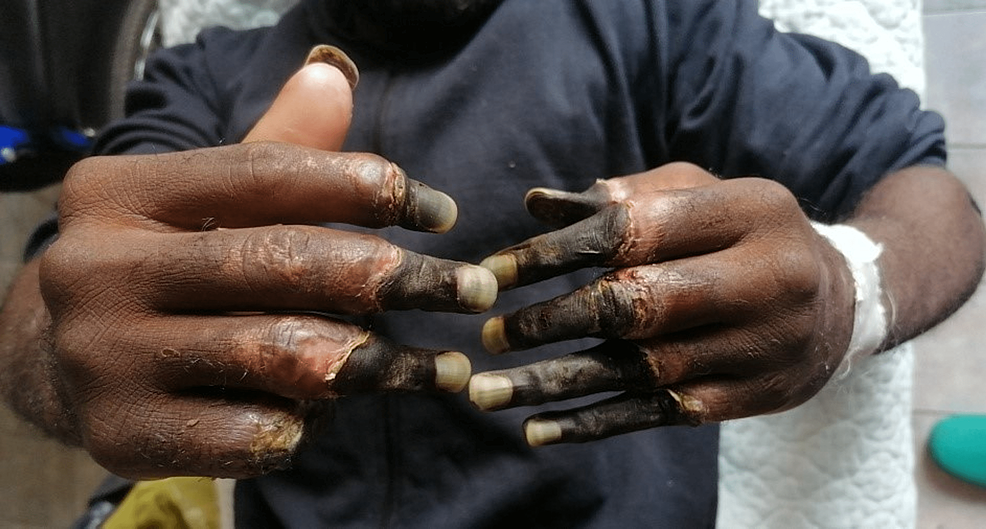The image depicts a close-up photograph of an African-American male, focusing predominantly on his severely damaged hands. He is presenting his hands palm-up towards the camera. Both hands display extensive frostbite damage: the fingers are blackened and shriveled from the knuckles down, with signs of gangrene evident in the tissue. The fingernails have turned black and white, indicating severe necrosis. Notably, the left hand is missing its pinky finger, and the remaining fingers appear heavily affected, with the tips showing a rotten black color contrasted by some white on the edges. The right hand still has a pinky, but the other fingers are similarly damaged. The man's wrists show a hint of white medical tape, possibly indicating prior medical treatment. He is dressed in a dark long-sleeve sweater, which contrasts against the white background, likely a wall or a cotton mattress. A teal shoe, likely worn by the person taking the photograph, is faintly visible at the bottom right corner of the image, corroborating the unusual angle, which suggests the man may be lying down.